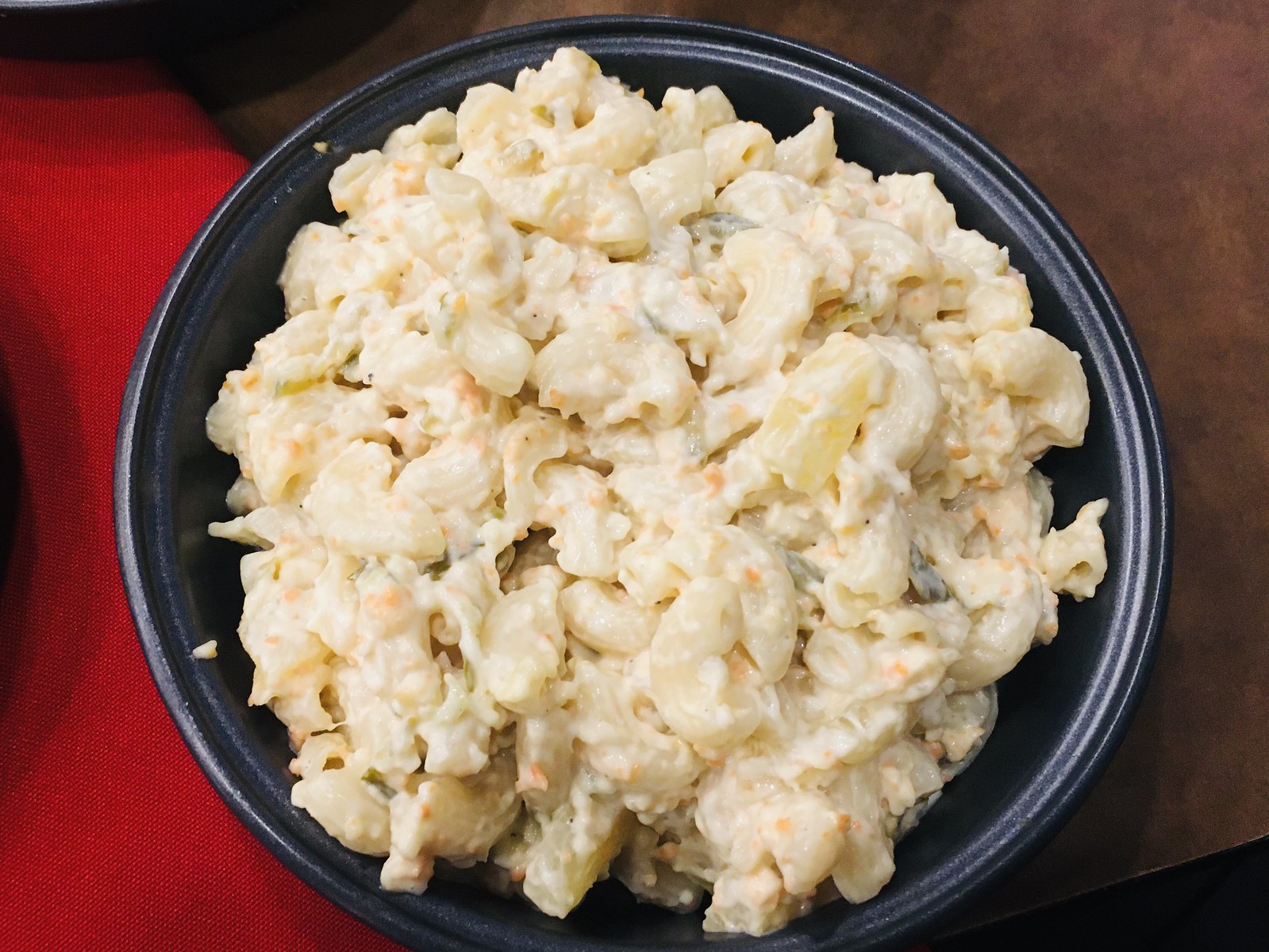The photograph captures a rectangular, wide-angle view of a black bowl filled with a creamy macaroni salad, centered prominently in the image. The bowl, with its recessed rim, sits on a brown surface speckled with black, which extends to the right side of the frame. To the left of the bowl, a red fabric napkin adds a splash of color. Within the bowl, elbow macaroni is generously coated in a white, possibly mayonnaise-based sauce, interspersed with tiny orange specks of grated carrot and occasional chunks of green vegetables. The composition is slightly asymmetrical, as the bottom portion of the bowl is cut off by the edge of the photograph, and the top right corner hints at the presence of another partially obscured bowl.